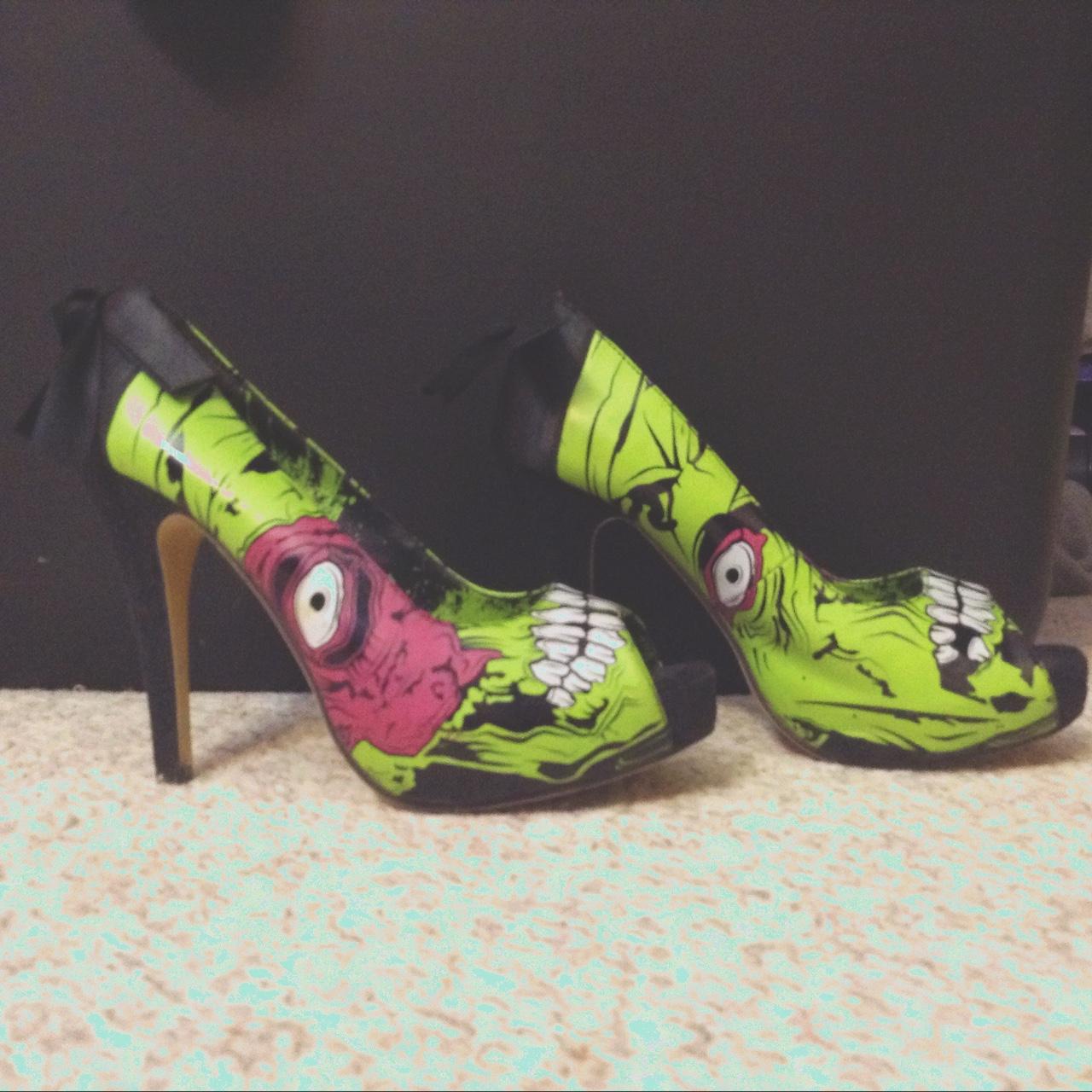This image showcases a pair of uniquely designed, custom-painted high heels set against a contrasting black background. The heels—each featuring approximately three-inch black stilettos and topped with shiny black ribbons—are placed side by side on what appears to be a marble table with a whitish-reddish hue. Each shoe displays an artistic rendering of a monstrous face, evoking a quirky, Halloween-themed style. The left shoe features an eye outlined in pink with a wide black iris, large white teeth near the toe, and vibrant pink and green hues. The right shoe mirrors this design but with subtle variations in the placement of the colors and details. The heels themselves are black, while the soles are a tannish color. Despite the somewhat blurry quality of the photograph, likely taken with an older camera phone, the vivid colors and distinctive monster face design stand out prominently, giving these high heels an eye-catching and whimsical appearance.